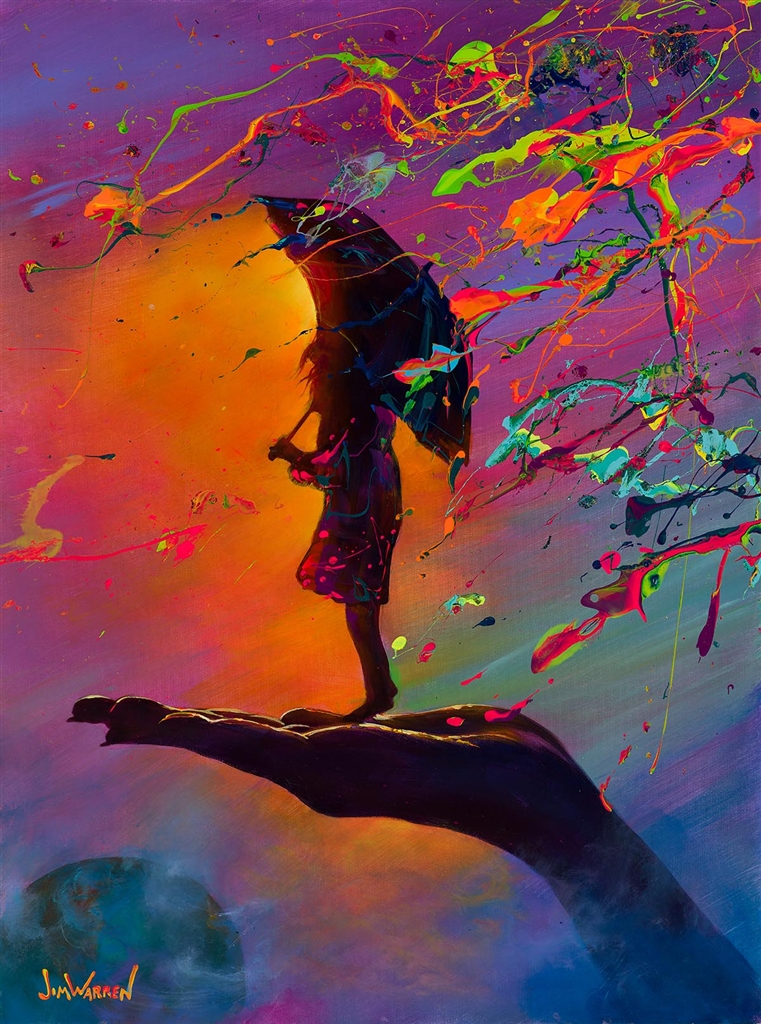This is a vibrantly colorful abstract painting, possibly hand-painted or computer-generated, depicting a silhouetted character held by a dark, shadowy left hand that occupies the bottom right of the canvas. The palm of the hand is facing up, with its fingers pointing to the left. Standing in the center of the hand is a silhouetted woman, mostly shaded in black with some hints of navy blue, wearing a purplish dark dress. She holds a black umbrella in her left hand, with its tip pointing upward and to the right, creating a protective arch above her head. Her long hair appears to be blowing in the wind toward the left.

The background transitions from an orange glow behind the character to streaks of purple that extend from the left and climb up to the right. The lower right corner features blue hues while the upper left is enveloped in more purple shades. Over this rich backdrop, splatters of paint in orange, green, red, and blue cascade from the top right, adding to the chaotic beauty of the scene.

In the bottom left corner of the painting, there is a prominent green sphere, possibly representing a moon, enveloped by a white wisp. Nearby, the artist's name, Jim Warren, is inscribed in exaggerated orange and yellow block letters, making it clear who created this fascinating piece. The overall composition merges dynamic elements of color and form, creating a visually arresting tableau.